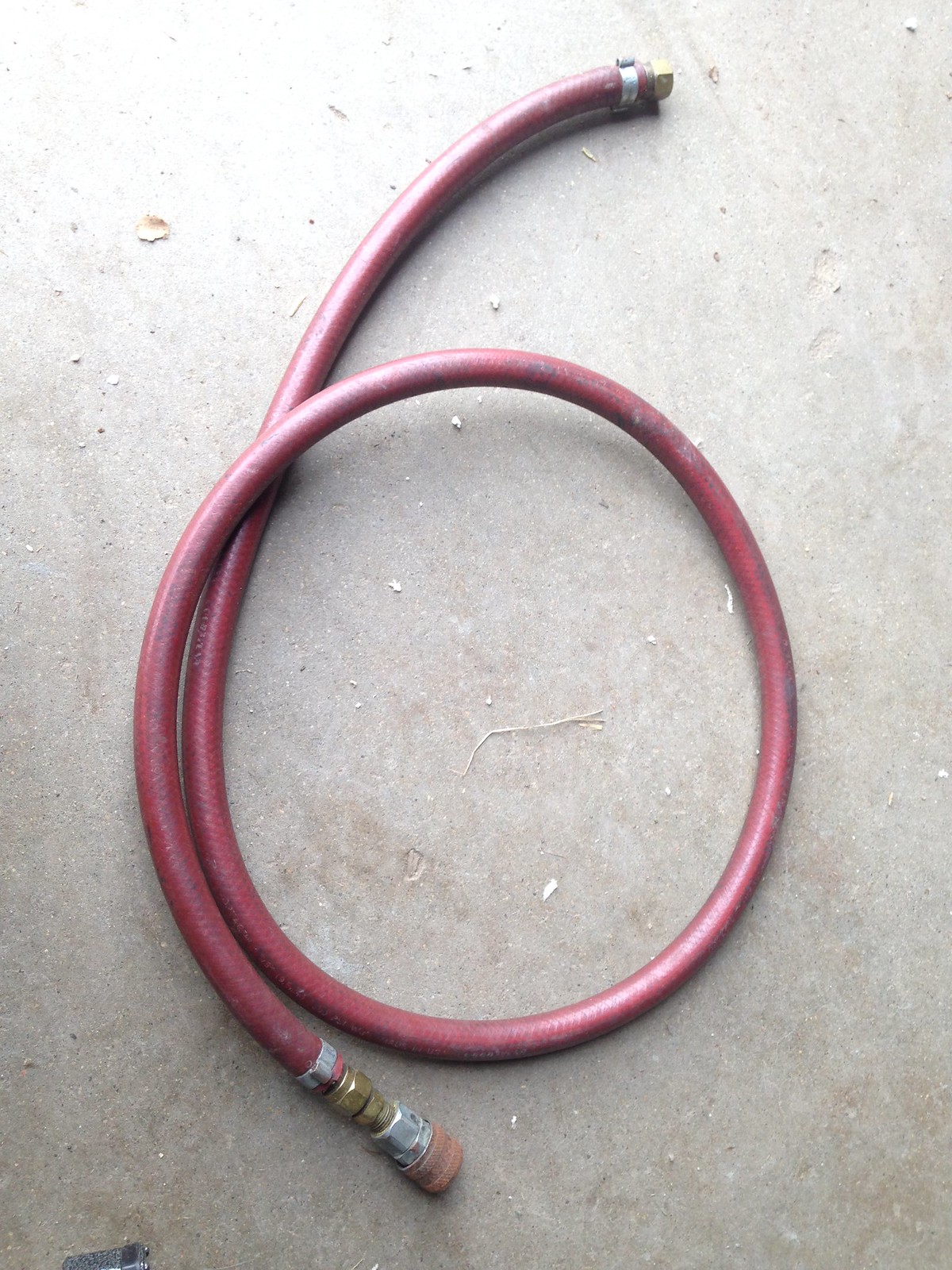This image showcases a red, coiled cable resembling the shape of the number six, laying on a mottled gray surface that appears to be concrete or asphalt. The concrete background is speckled with tiny pebbles and bits of dried grass or branches. The cable has dark red outer insulation and features metallic ends with brass and silver fittings, including washers, nuts, and crimping bands. The fittings at both ends are secured with silver clamps. The top right corner displays one end of the cable with an attached nut, while the bottom center reveals a detailed view of the other end, adorned with various metal components. Toward the bottom left of the image, there is a rectangular, silvery-gray box resembling a nine-volt battery lying on its side, identifiable by the two small bumps indicative of positive and negative terminals. The light catches the edges of the cable, highlighting its coiled structure and the slightly aged appearance of the metal fixtures, some of which show signs of rust.